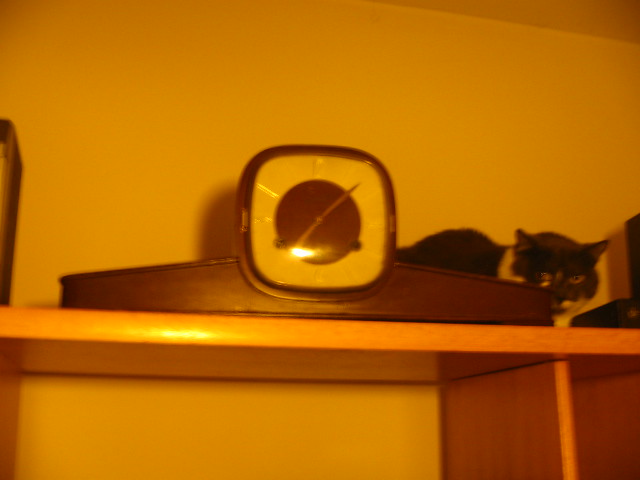A photograph captures a wooden shelf positioned high up near the ceiling, with the junction of the wall and ceiling clearly visible in the background. The central object on the shelf is a square-shaped clock with a long base, although the exact time is indiscernible due to a glare from a nearby light. Adjacent to the clock, a blackish-gray cat with white markings peers directly at the camera, giving the impression of hiding behind the timepiece. The intriguing placement and the curious gaze of the cat lend a whimsical charm to the scene.